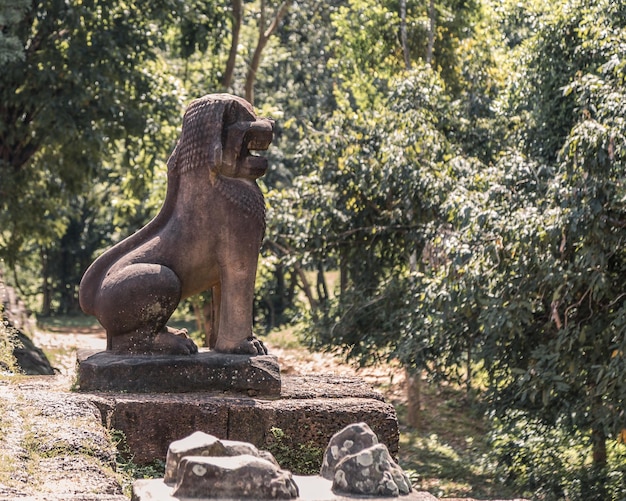The photograph, likely AI-generated, showcases an intriguing outdoor forest setting where one might feel they've discovered ancient ruins. At the center is a striking stone sculpture perched on a worn pediment, depicting an animal with an amalgam of features: the hind legs of a lion, the forelimbs and shoulders of a gorilla, and a face reminiscent of Fred Flintstone, complete with a set of white, human-like teeth. The statue’s mane appears almost braided. The creature is in a crouched position with a hint of a tail, yet no distinct tail can be seen. Adjacent to this sculpture, there's what remains of another statue—just the legs, suggesting it once stood alongside the current figure. Surrounding the sculptures is a forested area, vibrant with dense, out-of-focus foliage, creating a stark contrast with the clear, lichen-covered rocks in the foreground. The entire scene evokes a cultural landscape possibly reminiscent of Southeast or Southwest Asian temple grounds, emphasizing the mysterious and ancient ambiance of the setting.